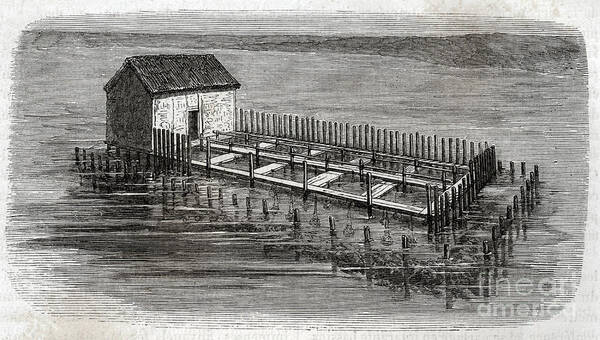The image is an older sketch, possibly from the 1800s, depicting a small house on stilts surrounded by water, which could be a lake, river, or part of the ocean. The house, featuring a dark gray rooftop and a small dark-colored door, is situated on a rectangular, frame-less plot with light-colored wooden stakes or posts protruding from the water. These stakes form a sort of fence that encircles the house, giving the impression of a defined boundary in the otherwise vast body of water. The water surrounding the house appears slightly gray, and some of the wooden posts seem to emerge from beneath its surface, hinting at a sunken or partially submerged structure. In the background, the water is segmented into smaller sections, resembling a water treatment plant or separated pools. The overall scene is rendered in black and white, capturing the rustic and mysterious nature of the setting.